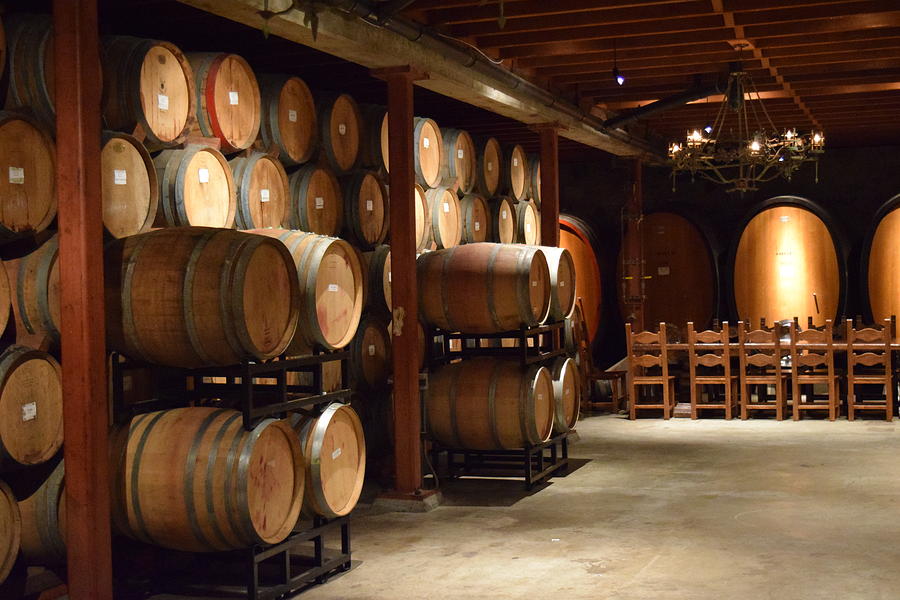The photograph depicts a contemporary warehouse, reminiscent of an Old West storage facility, with a concrete floor and a wooden-beamed ceiling. The left side of the image features numerous large wooden barrels, some of which are stacked in groups of four on metal shelves, arranged two-by-two on the bottom and top rows. Additional barrels are positioned behind these on separate racks, and there are several that stand alone, all of varying sizes.

In the background, a unique light fixture, devoid of glass and resembling a metal chandelier, hangs prominently from the ceiling, illuminating the space. Further back in the warehouse, there are even larger vats and a long dining table with a set of wooden chairs. On the side of the table facing away from the viewer, five chairs are visible, while additional chairs on the near side suggest a setup for a communal gathering or event. The photograph, taken in what appears to be a basement setting, encapsulates an intriguing blend of historical ambiance with a modern touch.